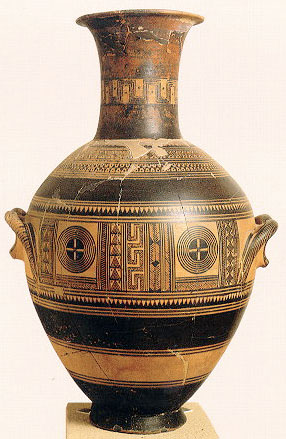This photo, likely taken inside a museum, features an ancient vase or urn perched on a concrete pedestal. The vase has a visually striking design, combining black and beige/gold hues. Its surface is oval-shaped with a narrow base, leading up to a funnel-like neck that widens slightly at the top. Noticeable cracks suggest it has been meticulously restored.

The bottom section of the vase displays alternating bands of black and beige/gold. Moving to the middle, the vase features intricate, horizontal designs accentuated by small grooved handles on either side. The decorations include concentric circles, columns resembling hieroglyphics, and circle-inside-square patterns. Towards the top, more bands of black and gold embellish the surface, with additional intricate designs between the stripes. Despite the visible cracks and minor chipping, the vase remains largely intact, indicating its significance and careful preservation, possibly as an ancient Egyptian artifact.